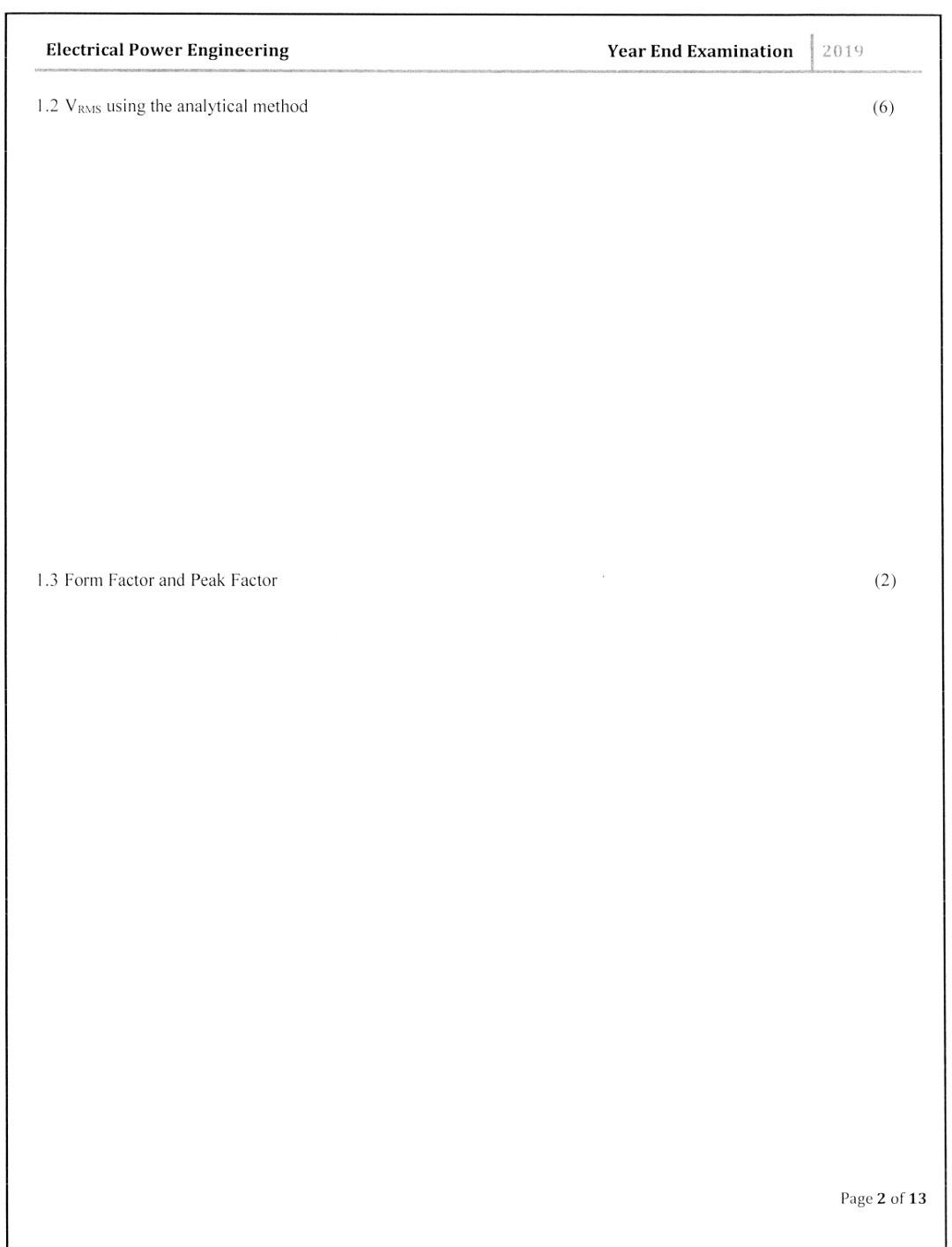This image depicts a page from a test or exam, specifically a Year-End Exam for the subject of Electrical Power Engineering dated 2019. The page has a black border that outlines the top, left, and right sides but is open at the bottom. At the bottom right corner, it is marked "page 2 of 13," where the numbers "2" and "13" are in bold black font, while the words "page" and "of" are in a regular font.

At the top of the page, the title "Electrical Power Engineering" is written in bold on the left, and on the right, also in bold, is "Year End Exam." This section is underlined by a thin gray line with the year "2019" printed in a lighter gray just above it. Below the top header, the following problems are listed:
- "1.2 VRMS" with RMS in subscript, accompanied by the instruction to use the analytical method, and a "6" in parentheses on the far right.
- "1.3 Form factor and peak factor" with a "2" in parentheses also on the far right.

This provides a structured and detailed visual context, indicating that the document belongs to the second page of a comprehensive exam.